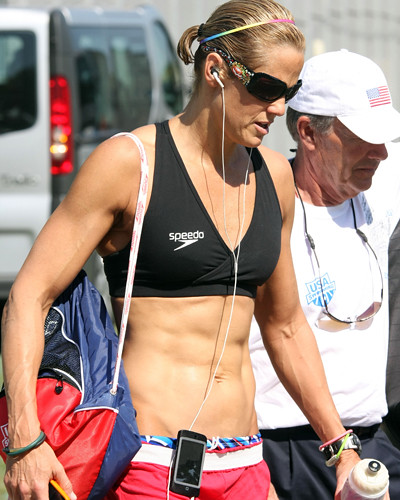In this vivid daytime outdoor image, we see a variety of elements coming together to create a dynamic scene. The background features a concrete or stone wall, and in the upper left corner, there are a couple of cars parked, suggesting a possible parking lot setting. It's sunny and very bright, enhancing the details and colors in the photograph.

At the center of the image, a man and a woman are captured while walking together. The woman stands out with her athletic appearance; she has blonde hair, wears a black pair of sunglasses, and has headphones in. Her outfit consists of a bikini top with the brand "Speedo" visible, paired with pink shorts. She also carries a water bottle, has a fitness watch on her wrist, and looks very fit and toned.

Accompanying her to the right is an older man, donning a white hat emblazoned with the American flag, a white shirt with "USA" printed on it, and gray shorts. The detailed portrayal of their attire and accessories, combined with the bright and clear weather, captures the essence of an active, sun-soaked day, likely spent near the beach or in a similar relaxed outdoor environment. The blend of grays, browns, yellows, blues, reds, and other rich colors contribute to the detailed and lively depiction of this moment.